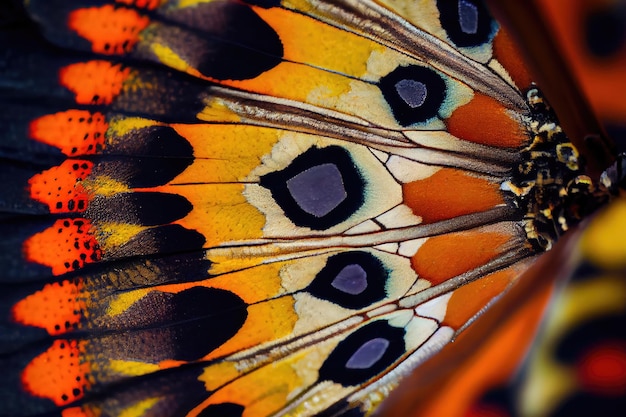This highly detailed, close-up photograph captures a vibrant section of a butterfly's wing, filling approximately a third of the frame. The wing features a stunning array of colors, including vivid oranges, blacks, yellows, blues, whites, and cream, meticulously segmented into distinct areas by fine veining. Each segment showcases elaborate patterns, such as a black oval with a blue center reminiscent of an eye, gold patches, and asymmetrical sections of rust and white. Small dots of orange and additional black segments add to the intricate design. The background is blurred, highlighting the wing's exquisite detail and the texture of the fine scales. The image is zoomed in so closely that it likely required a specialized camera to capture such rich detail, as a standard camera or phone wouldn't suffice. Though it's ambiguous whether the scene is indoors or outdoors, the striking combination of colors and patterns suggests an exotic natural environment, possibly hinting at the butterfly's unique transformational beauty on the right edge of the wing.